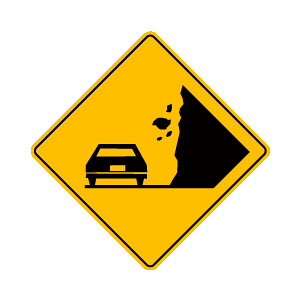This is an image of a road sign set against a plain white background. The sign is diamond-shaped and features a yellow background with black symbols. On the left side of the sign, there is an icon of a car. On the right side, a triangular black shape represents a steep cliff or mountainside from which numerous black blobs appear to be falling. These falling blobs symbolically indicate potential falling rocks on the road, warning drivers of the danger ahead.